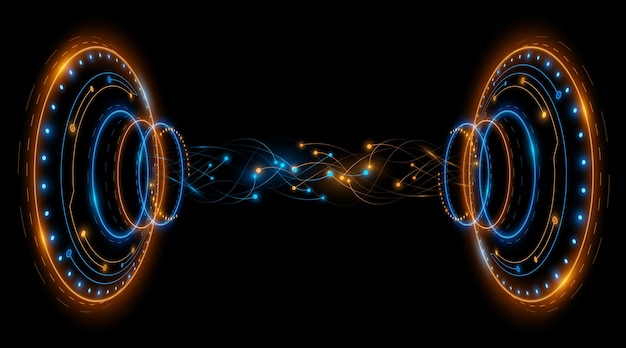The image features a predominantly black background with a striking, almost symmetrical design centered on two circular structures facing each other. Each structure is composed of concentric rings with distinct colors and patterns. Starting from the outermost ring, there's a golden-bronze circular ring, followed by an inner circle of blue dots. This pattern repeats with alternating blue and gold rings, creating a layered, vibrant effect. Both circular structures emanate light, with blue lights jutting out from the left structure and orange lights from the right. Within these circles, there are also smaller dots with tails, creating an electrified appearance. The central region between the circles seems to emit energy, further emphasizing the dynamic, almost three-dimensional feel of the entire image. The design employs a limited color palette of blue, orange, and gold, enhancing its visual impact.